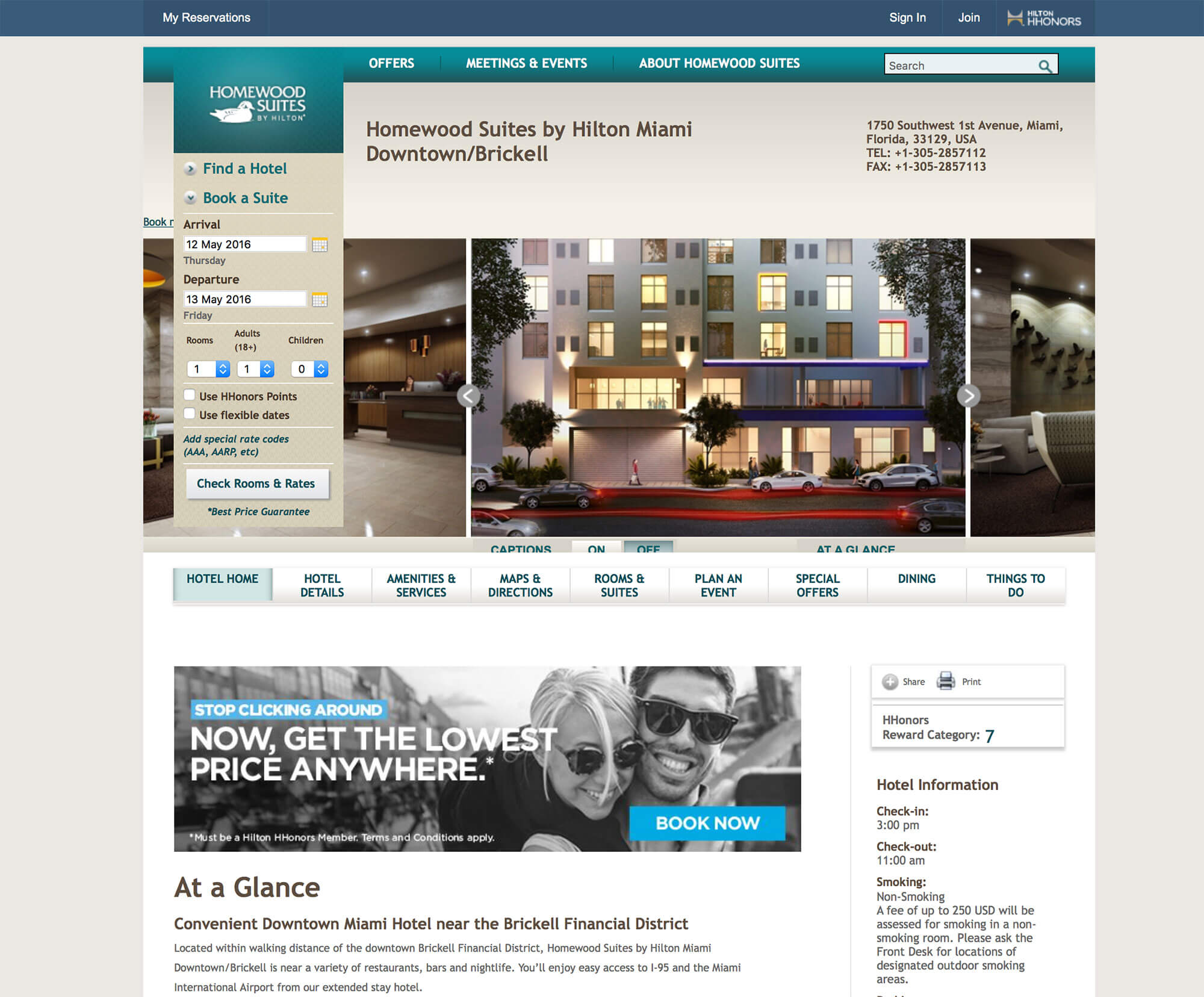This screenshot depicts a webpage for Homewood Suites by Hilton, specifically the Miami Downtown Brickell location. The user has conducted a search for a stay at this hotel in Miami, arriving on May 12, 2018, and departing on May 13, 2018, for one adult. The webpage prominently features the hotel's name and address: 1750 Southwest First Avenue, Miami, Florida, 33139, along with contact information including a telephone number and a fax number.

The page displays images of the hotel's lobby, exterior, and several interior areas to provide a visual representation of the accommodations. Lower on the page, there are multiple navigation headers, including Hotel Home, Hotel Details, Amenities and Services, Maps and Directions, Rooms and Suites, Plan an Event, Special Offers, Dining, and Things to Do.

Additionally, the webpage provides essential information such as check-in and check-out times (3 p.m. and 11 a.m., respectively), adherence to a non-smoking policy, and a brief summary highlighting the hotel's convenient location near the Brickell Financial District in downtown Miami.

The final step for the user to see the room rates and availability would be to click the "Check Rooms and Rates" button, guiding them towards securing their reservation.